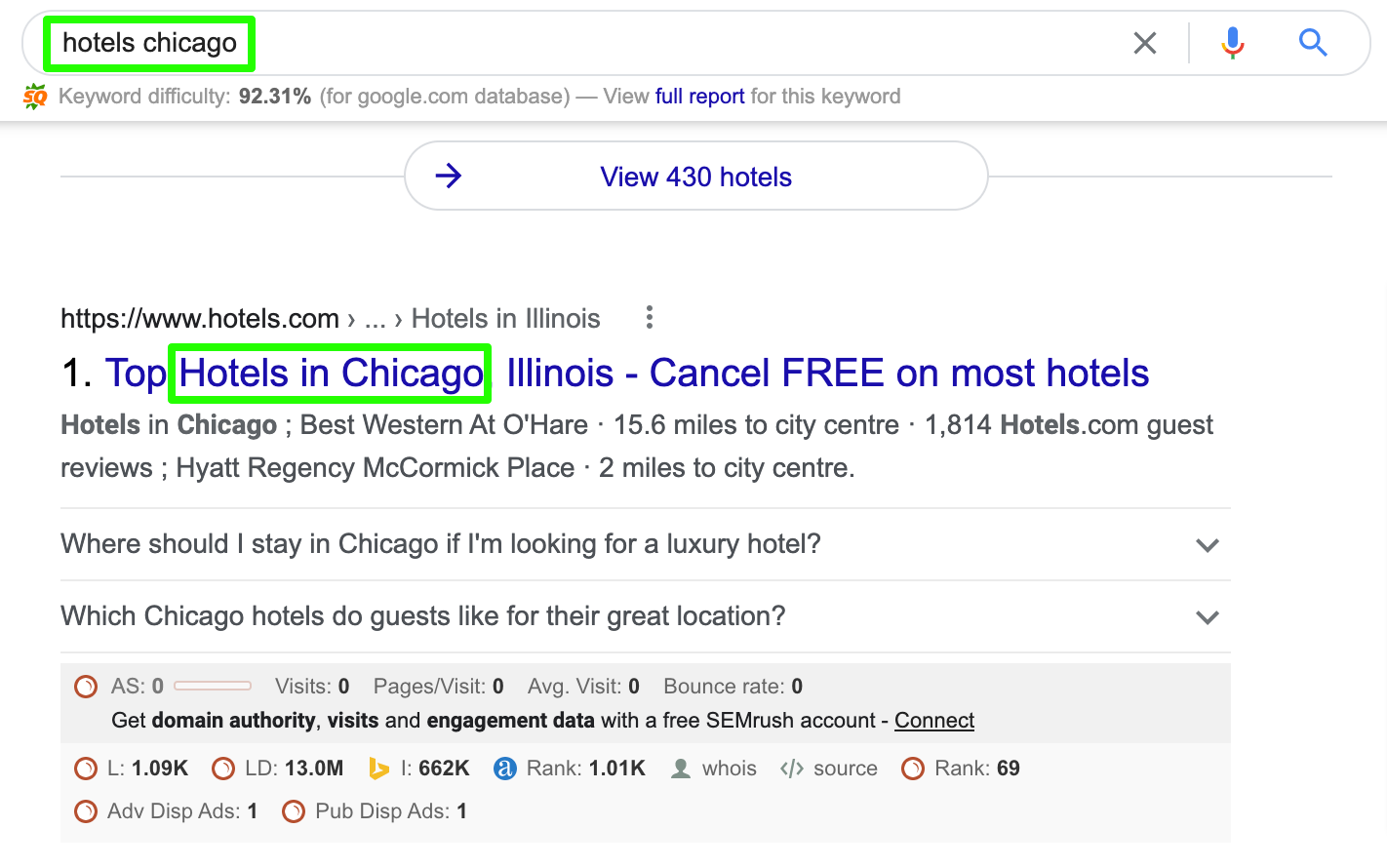The screenshot displays a desktop view of Google Analytics focused on the search term "hotel Chicago." A search box at the top highlights the entered keyword, with a keyword search difficulty of 92.31% for the google.com database indicated just below.

Beneath this, a blue link prompts users to "view 430 hotels," leading to a search result from hotels.com. The search result's title reads "Top Hotels in Chicago, Illinois - Cancel Free on Most Hotels." It lists individual hotels such as "Best Western at O'Hare," located 15.6 miles from the city center, and "Hyatt Regency McCormick Place," located two miles from the city center. Guest reviews from hotels.com indicate 1,414 reviews for the Best Western.

Two notable questions follow the listing: "Where should I stay in Chicago if I'm looking for a luxury hotel?" and "Which Chicago hotels do guests like for their great location?" Further below, the screenshot reveals more analytics and various numerical data.